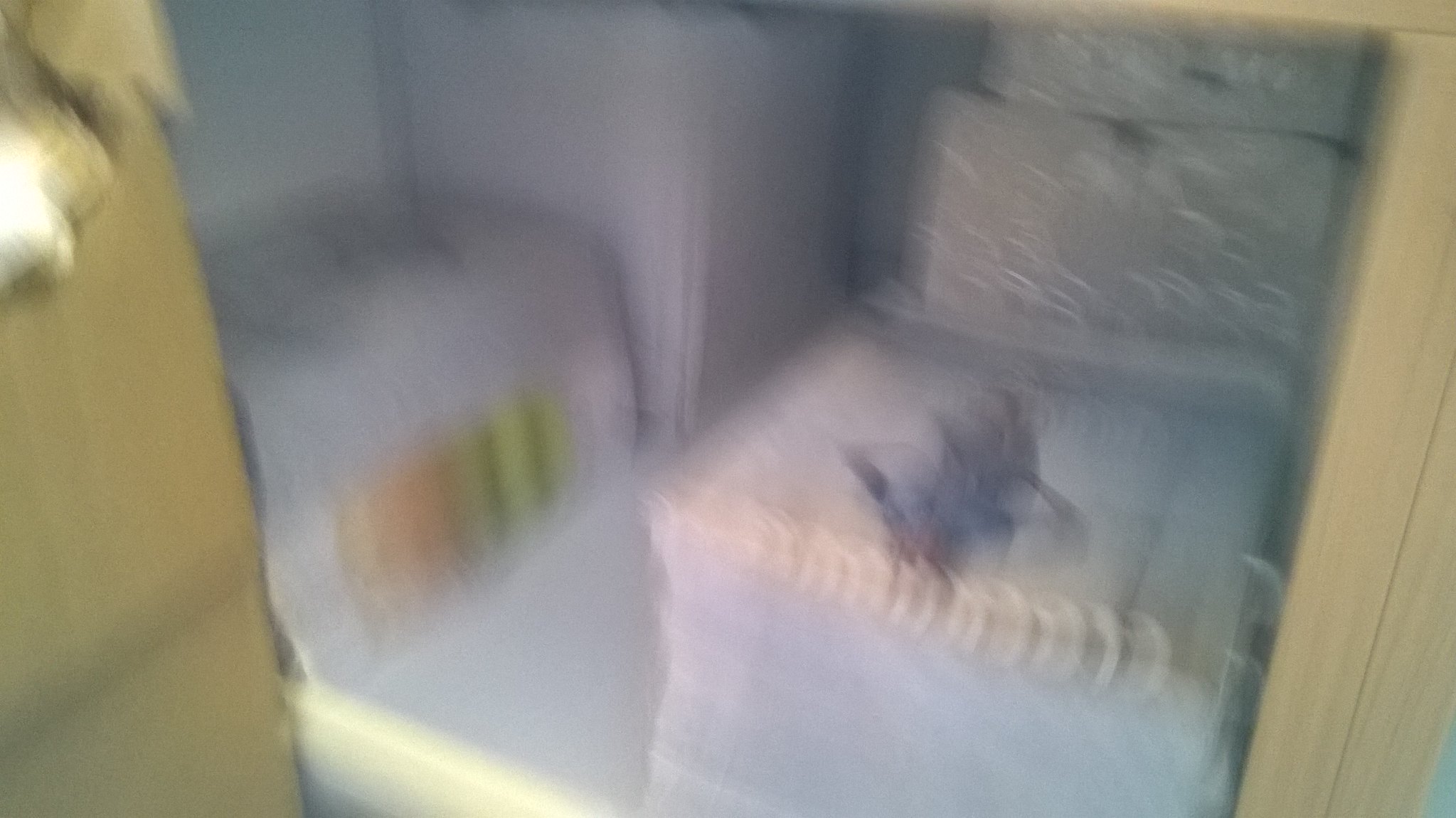The extremely blurry image appears to depict a small space, possibly a closet or laundry room. In the back left corner, a taller appliance, potentially a washing machine, is vaguely visible. To its right, two ottomans are discernible, each stacked with what seem to be soft blue blocks or towels. Atop one ottoman, there appears to be a small, plush, blue toy bird. Further to the right, additional blue boxes with distinguishing orange and green striped squares on the sides can be seen. The bottom left of the image shows the side of a brown cardboard box with a yellow circle near the top, and its upper left corner appears frayed or ripped. Wooden framing is evident around the outer edges, forming a light brown structure that partially frames the scene. Despite the blurriness, the image conveys a space cluttered with various indistinct items, all set against a gray ground.